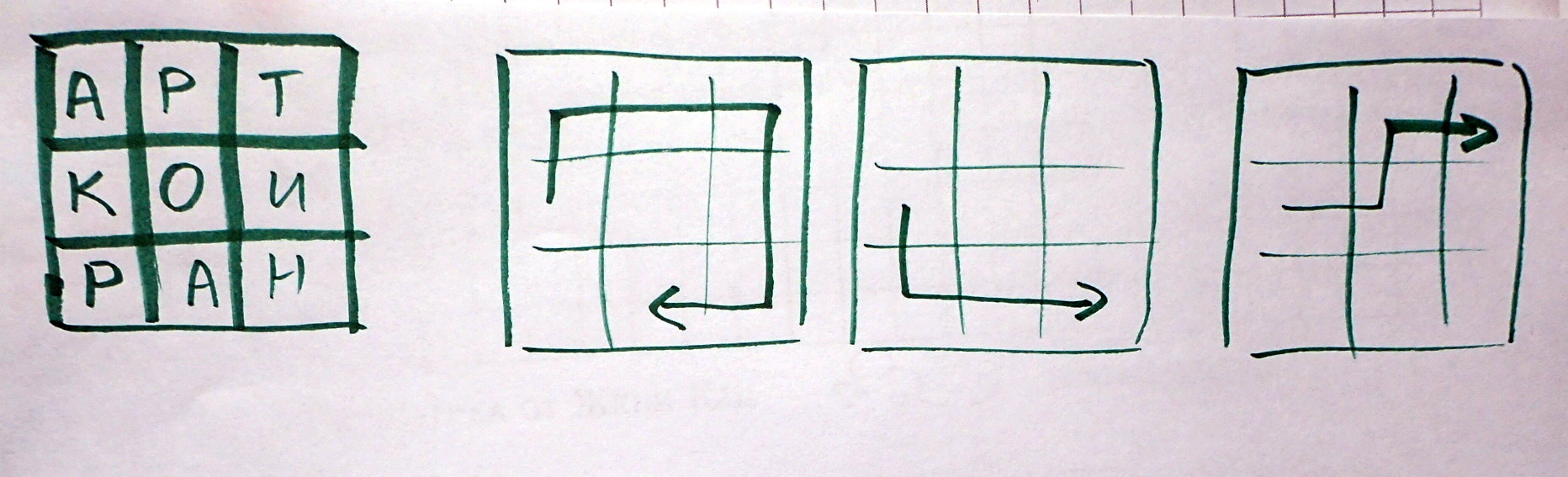The image above contains four distinct squares, each featuring unique outlines and designs:

1. **First Square**: This square is configured like a tic-tac-toe game board, divided into nine smaller cells arranged in a 3x3 grid. Within these cells, letters are positioned sequentially from left to right and top to bottom. The top row contains "A," "P," and "T." The middle row consists of "K," "O," and "U." The bottom row is filled with "P," "A," and "H."

2. **Second Square**: Similar in layout to the first, this square is also divided into a 3x3 grid. However, within the larger outer square, there is an additional shape resembling more than half of another square with an arrow. This arrow is oriented to the left when facing the image, adding a dynamic contrast to the grid design.

3. **Third Square**: Again featuring a 3x3 grid, this square mimics the layout of the second square but with a notable variation in the inner shape. This time, the arrow-like feature is not as extensive and points to the right, creating a mirrored effect relative to the second square.

4. **Fourth Square**: The details of the fourth square are not fully described, but it is implied that it could contain another variation or design complementary to the first three squares.

Overall, these four squares showcase a combination of grid-based and dynamic, arrow-laden designs, merging structured and fluid elements within a single cohesive image.